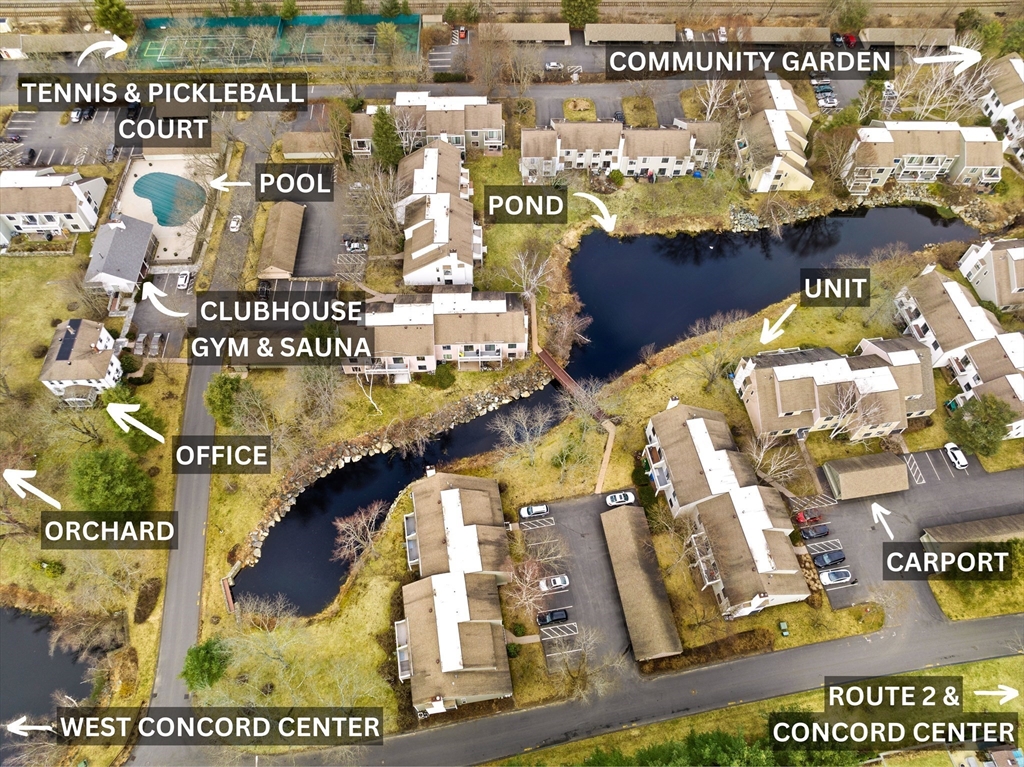A digitally enhanced, full-color aerial photograph vividly depicts a meticulously planned community or apartment complex. Captured from above, this square image, devoid of any borders or background, showcases various labeled amenities and buildings. Dominating the scene are numerous white buildings with light brown roofs, surrounded by sprawling green spaces and blacktop parking lots, all hinting at a fall setting given the bare trees except for some verdant pine trees.

Prominently, a deep blue pond with a rocky wall is centrally located, enhancing the picturesque environment. The labels, which include small illustrative icons, clearly identify key features: the upper left corner highlights tennis and pickleball courts, while the upper right marks a community garden. The center of the image is dedicated to the pond, encircled by units. Additional labels guide the viewer to a pool, a clubhouse, a gym and sauna, office spaces, and an orchard, all situated within the complex. Notably, arrows connect these labels to their respective structures, providing a comprehensive map-like overview. The right side of the image features labels for a unit, carport, Route 2, and Concord Center, tying the complex to its surrounding area and emphasizing its well-organized layout.